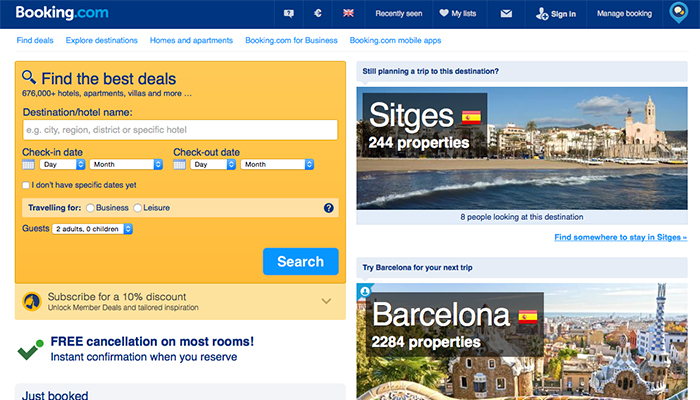Screenshot from the website Booking.com.

The top quadrant features a dark blue horizontal bar with the text "Booking.com" prominently displayed. The word "Booking" is in white, while ".com" is in blue. On the right side of this bar, there are several navigation hyperlinks, though the functions of the first three are unclear due to their small size. The fourth hyperlink reads "Recently Seen," followed by one with a heart icon labeled "My List." Next are icons for email, account sign-in, managing bookings, and a chat feature.

Beneath this dark blue strip, additional navigation hyperlinks appear in blue text on a white background. They read: "Find Deals," "Explore Destinations," "Homes and Apartments," "Booking.com for Business," and "Booking.com Mobile Apps."

In the center-left area of the screen, there is an orange or goldenrod box featuring a search field for finding the best deals among over 676,000 hotels, apartments, villas, and more. Users can search by destination, hotel name, check-in and check-out dates, with an option to specify flexible dates, type of travel (business or leisure), and number of guests.

Below this, another box offers a subscription for a 10% discount, unlocking member deals and tailored inspiration.

To the right of this is a box with a bluish background, prompting users who are still planning a trip to Sitges. It mentions there are 244 properties available and includes an image of a beachfront villa with a note that eight people are currently looking at this destination. A hyperlink below encourages users to "Find somewhere to stay in Sitges."

Further down, another promotional box suggests trying Barcelona for a future trip, featuring an image of Barcelona's city center. It mentions there are 2,284 properties available in Barcelona and includes a darker overlay.

In the bottom left corner, a hyperlink promises free cancellation on most rooms, instant confirmation upon reservation, and highlights recently booked properties.

The overall background of the website is white, providing a clean and organized look to the layout.